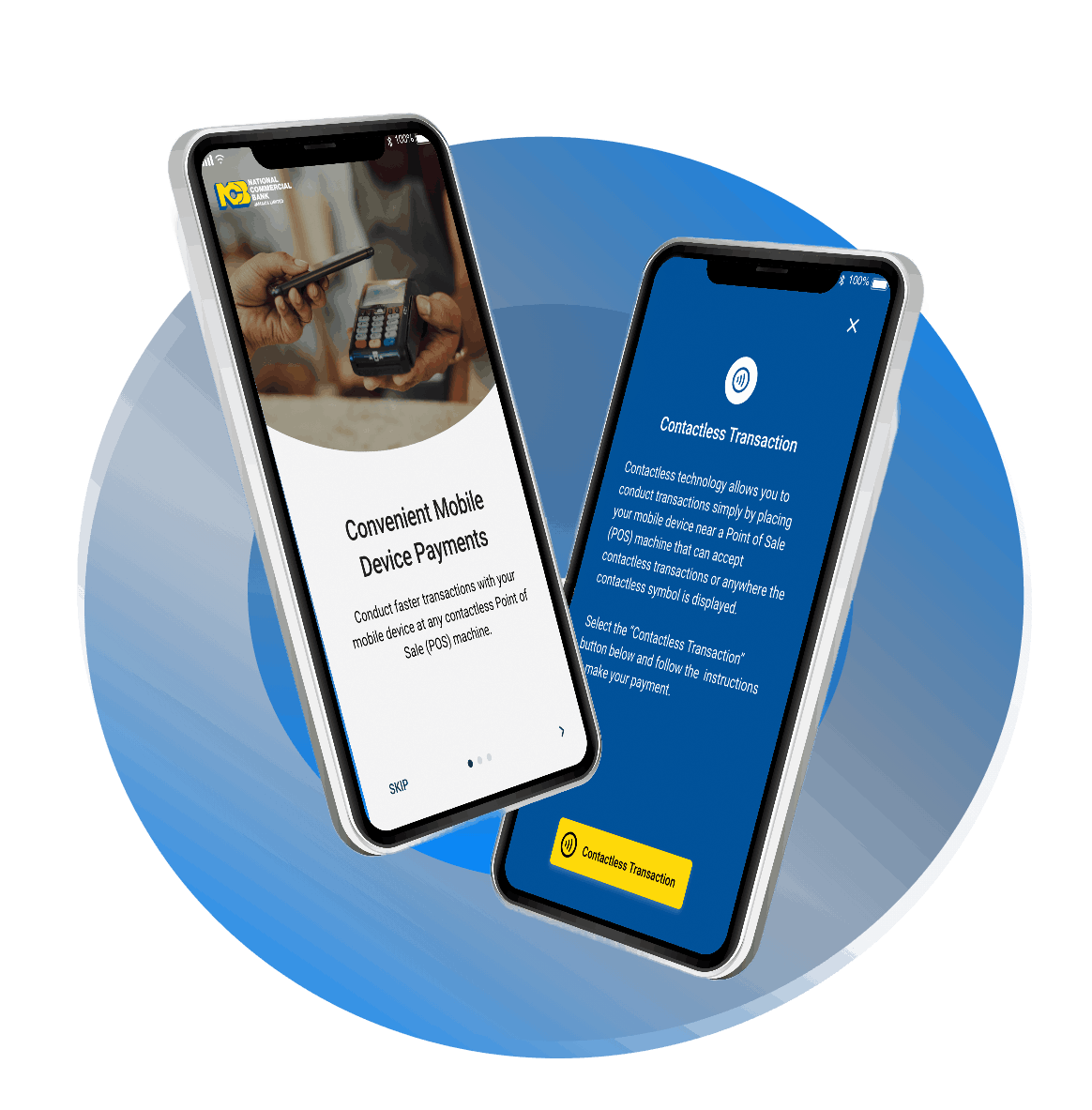A promotional screenshot advertising mobile payment devices features a predominantly blue circular gradient background, transitioning from a darker hue in the upper right to a lighter hue in the bottom left. Central to the image are two gray smartphones with black screens, set against the blue backdrop. The left device depicts a hand holding a generic black smartphone towards the center, while the right device features a hand presenting a black card reader ready for a credit card transaction.

Beneath the graphic, there is text on a white background that reads, "Convenient mobile device payments," though the design appears unpolished. An additional block of text states, "Conduct faster transactions with your mobile device at any point of sale (POS) machine." To the right of the devices, in a blue section with white text, further details are provided: "Contactless transaction. Contactless technology allows you to conduct transactions simply by placing your mobile device at a point of sale (POS) machine that accepts contactless payments or anywhere the contactless symbol is displayed."

At the bottom of the image, a yellow rectangle with black text emphasizes the main theme with the phrase "Contactless transaction." The overall presentation suggests a focus on the ease and speed of mobile payments using contactless technology, despite the amateurish design execution.